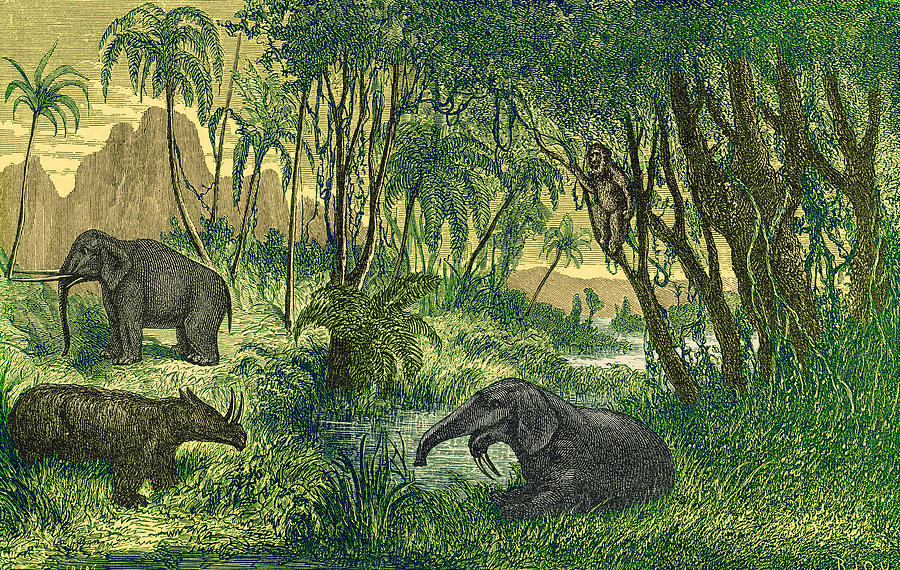The image depicts a detailed, portrait-mode artistic rendition of a lush jungle scene, akin to a wood carving or a sketch, evoking a naturalistic style reminiscent of murals at the Museum of Natural History. The sky, situated in the upper left-hand corner, is rendered in creamy tan hues. Below, two towering palm trees are set against a backdrop of numerous densely leaved and trunked trees, extending down to grassy terrain, with greens and yellows marking the foliage.

In the foreground, grassy patches appear in both the left and right bottom corners, accentuating the earthy ambiance. A series of vines hang from the trees, contributing to the overgrown aesthetic. Prominently at the center of the bottom half, one elephant is seen reclining by the water, its tusks pointing downward with its trunk curving upward. Above this peaceful pachyderm, a monkey lounges in the trees, presiding over the scene below.

To the left of the reclining elephant, a rhinoceros-like creature—dark in color and featuring bones resembling tusks protruding from its nose—adds to the exotic fauna. There is also a second elephant, depicted in a natural gray tone and facing to the left, contributing to the vibrant wildlife imagery. The background is completed with distant mountains, enhancing the depth of this richly detailed environment.

The art piece includes the initials "RJOV" and some barely legible numbers at the very bottom, further grounding this intricate portrayal of the jungle's lively ecosystem.